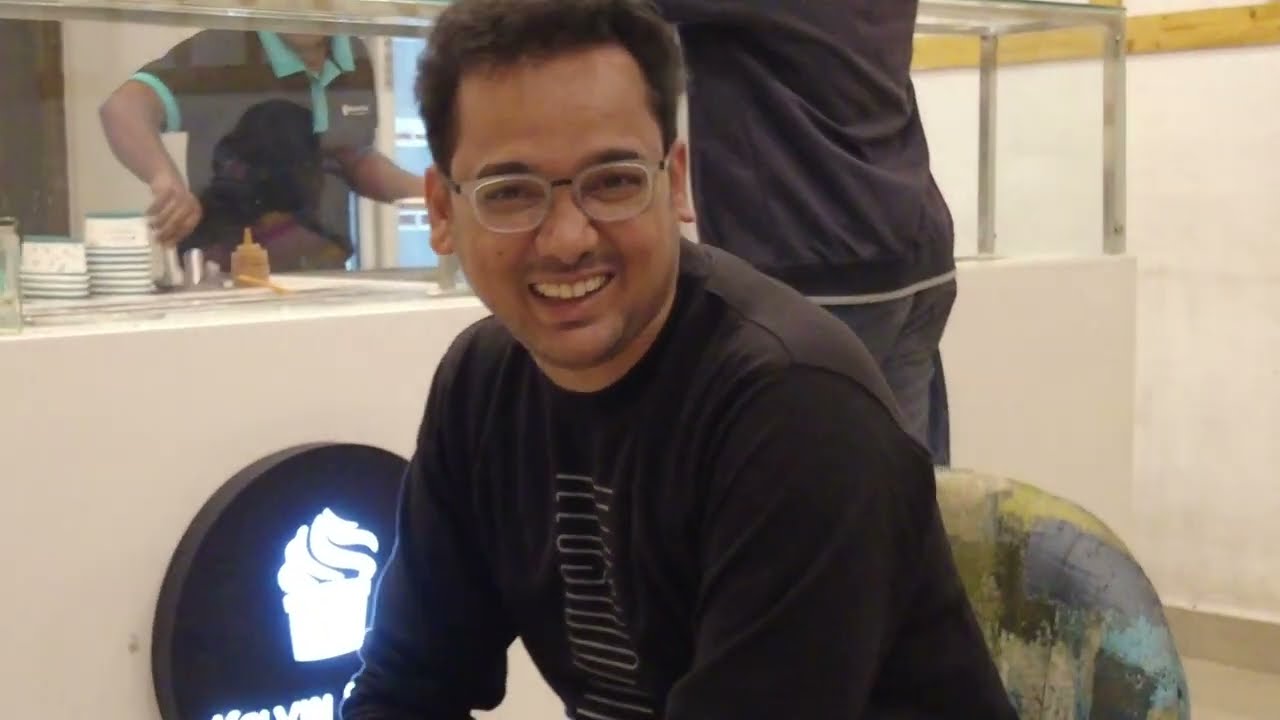In the image, there is a young man with short, dark brown hair and a receding hairline, smiling and leaning forward in the foreground. He is dressed in a black long-sleeved shirt and wearing small, ovular, clear glasses. He has a stubble and appears to be seated on a chair with a multicolored print.

Behind him is an ice cream parlor counter with a glass window. Embedded in the counter is a circular, black logo approximately three feet in diameter, illuminated with an LED light in the shape of a cupcake. Behind the counter, a man, who appears of possibly Spanish descent and has darker but not black skin, is wearing a dark navy blue button-up shirt with light blue linings on the sleeves. He is scooping ice cream to serve a customer.

The customer in front of the counter, partly visible from the back, is wearing a black hoodie and gray pants. The overall scene suggests a cheerful and busy atmosphere within the ice cream parlor.